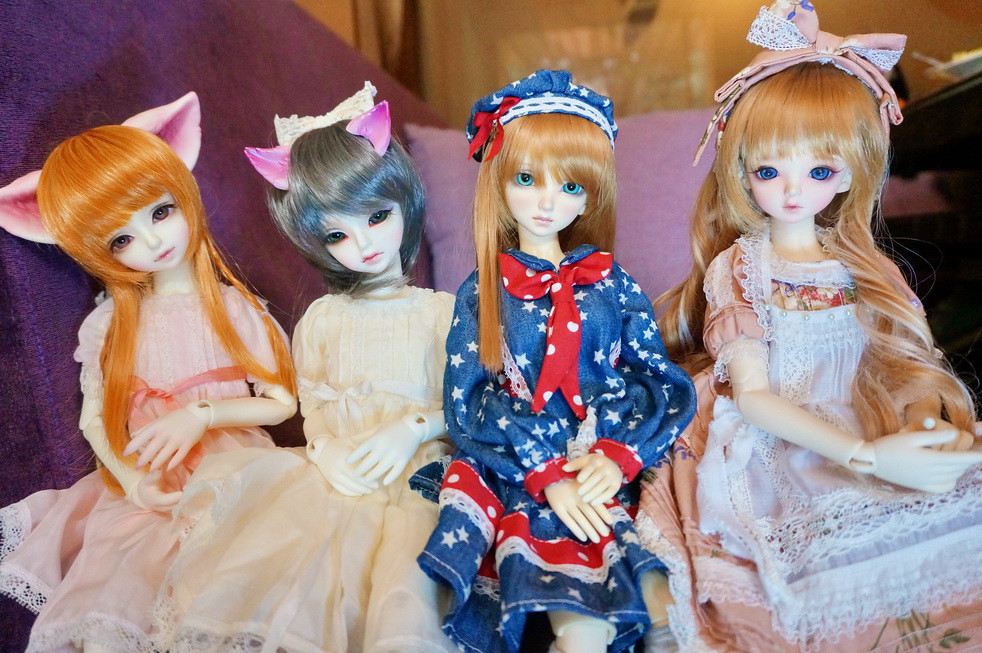The photograph features four dolls seated side by side on a purplish couch against a brown wooden wall. Accompanying the dolls, there is a lighter pink pillow on the couch. The first doll on the far left has long orange hair with fringe and pink, cat-shaped ears on top of her head. She is dressed in a light pink dress. The second doll features short, chin-length gray hair and pink cat ears, donning a white dress. The third doll has long blonde hair that cascades towards her back and sports an American-styled red, white, and blue dress with white stars and red trim. The final doll on the far right has extremely long blonde hair reaching down to her hips and wears a pink dress with a white apron, complemented by a pink bow in her hair. All the dolls have fair skin and distinctively large eyes, each adding to their charming appearance.